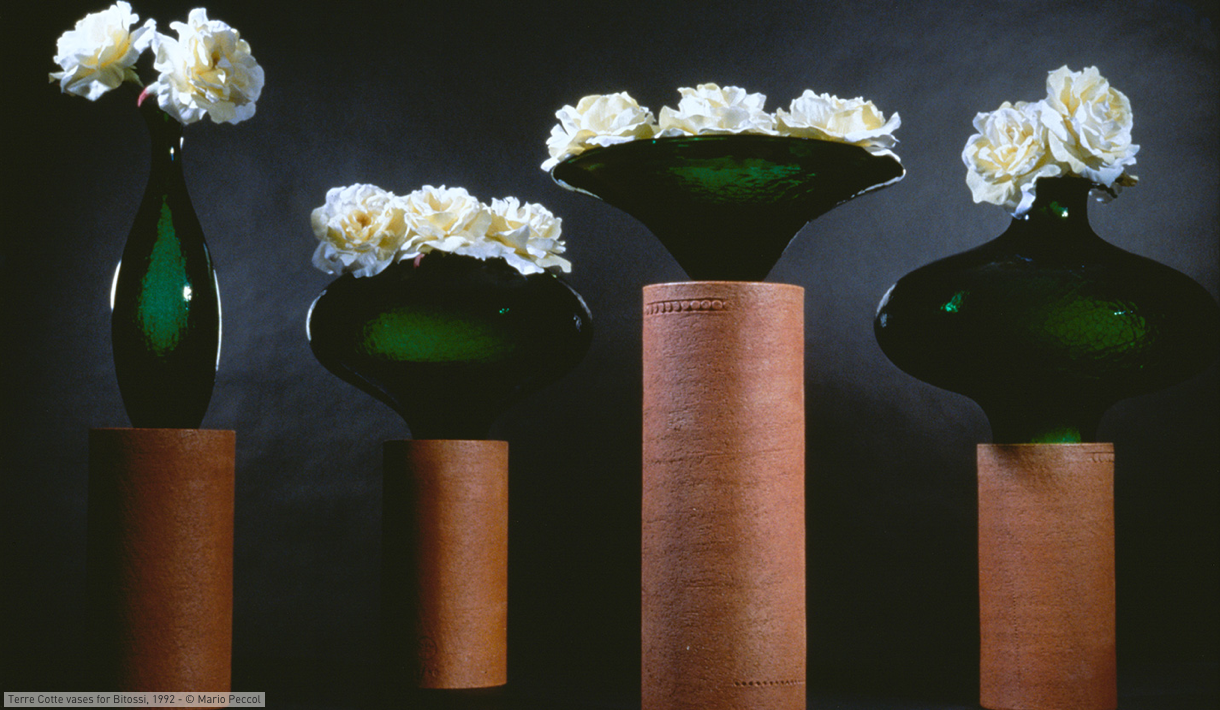The photograph showcases four distinct green vases, each adorned with white flowers and resting on cylindrical, orange-brown stands. From left to right:

1. The first vase is tall and slender, holding two white flowers.
2. The second vase has a bulbous, tear-shaped design, containing three white flowers.
3. The third vase is wide and shallow, resembling a bowl or dish, with three white flowers.
4. The fourth vase tapers at the top after a bulbous bottom, also holding two white flowers.

Set against a nearly black or dark gray background, the image has an elegant and striking contrast. In the bottom left corner, the text reads, "Terracotta Vases for Betosy 1992, copyright Mario Pekel."